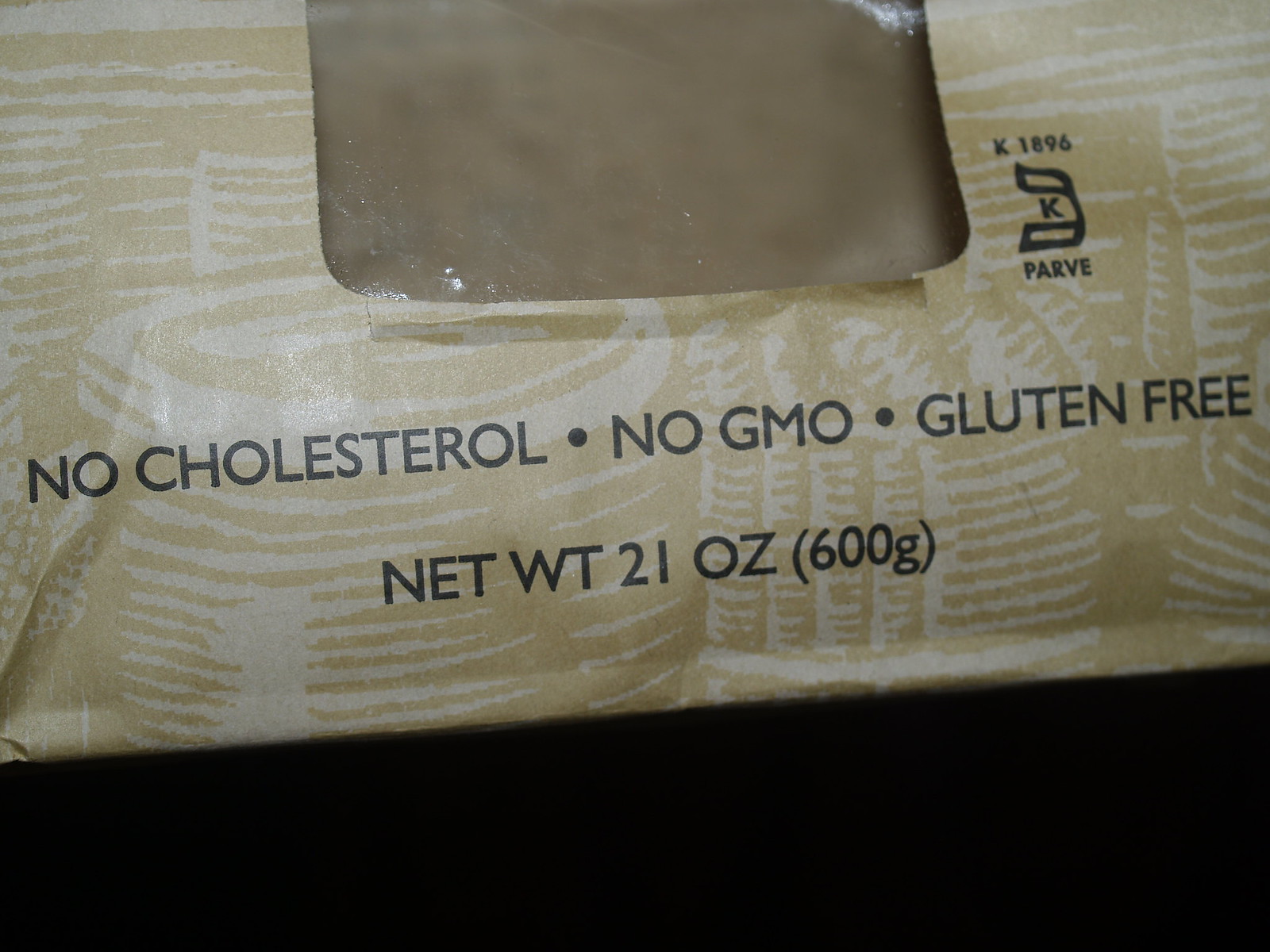The image depicts a close-up, cropped view of the bottom part of a bread package, photographed against a black background. The packaging, made of brown and beige paper, features a wood and barrel motif with striped lines. Central to the image is a rounded rectangular cut-out, covered with clear cellophane, through which a darker brown material is visible. In black print along the bottom of the package, it reads "no cholesterol," "no GMO," and "gluten-free," with black dots separating each phrase. Below this, it states the net weight of the item as 21 ounces (600 grams), and there's an additional symbol to the lower right near the viewing window, featuring a "K" in a circle with "PARVE" written below and "K1896" above. The horizontal orientation of the photograph captures about three-quarters of the package, with the black background filling the remainder of the frame.